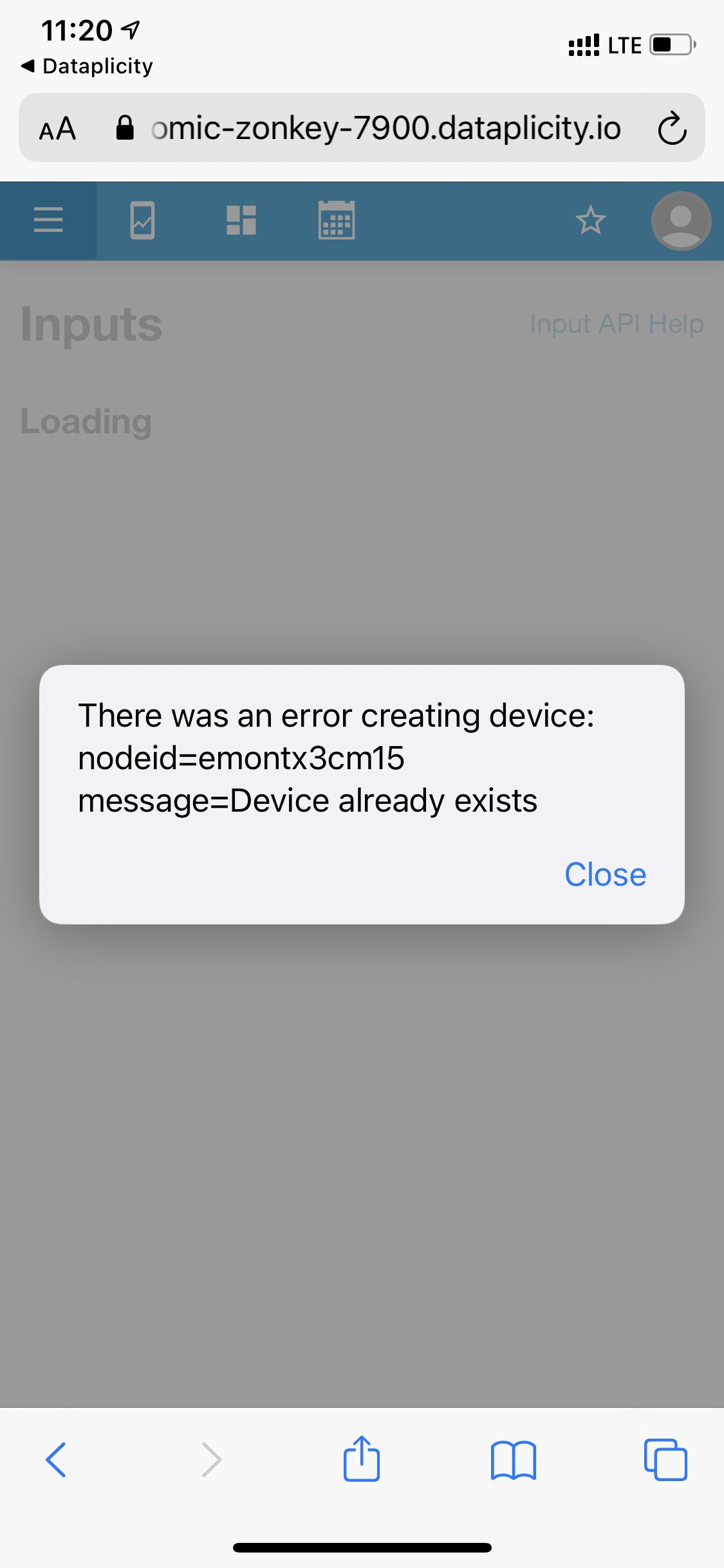This image is a screenshot from a smartphone. The top border of the screen is a very light gray color. On the top left, the time "11:20" is displayed in black font. Directly beneath the time, the word "Dataplicity" is visible. To the left of "Dataplicity," there is a black rectangle pointing to the left, which likely represents a back button. In the upper right corner, the battery icon shows approximately half charge. Next to the battery icon, "LTE" is written in capital letters, indicating the type of wireless connection.

The screenshot partially reveals a website address: "OMIC-zonkey-7900.dataplicity.io." Below this, the top border of the webpage is blue, and the background is gray. The webpage displays the words "Inputs" with "Loading" beneath it on the left side.

In the center of the screen, there is a white rectangle with rounded edges. Inside this rectangle, a medium gray font states, "There was an error creating device." Following this message, a string "nodeid=emontx3cm15" is displayed, along with another message that says "message=device already exists."

In the lower right corner, "Close" is written in blue font, most likely a button to dismiss the error message.